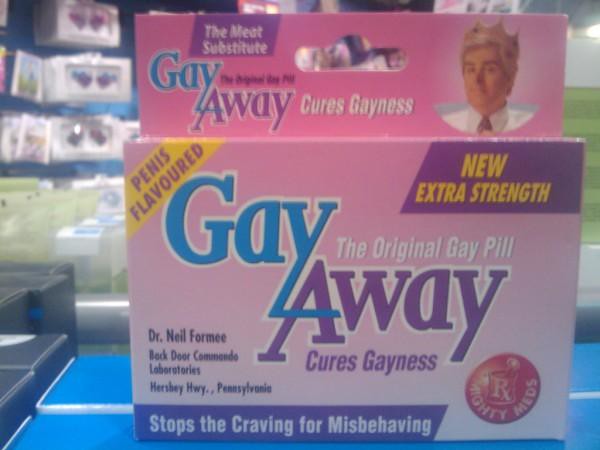This detailed color photograph captures a satirical product prominently displayed in what appears to be an indoor setting, possibly a prank or novelty store. The product, a box of tablets, is centrally positioned atop a shelf or counter, with other items faintly visible in the background.

The packaging is primarily pink with blue and purple lettering, giving it a vibrant and eye-catching appearance. The top right corner features a small image of a Caucasian male with blonde hair, a golden crown, a fake tan, and a buttoned-up white dress shirt, adding to the comedic effect of the product. 

The product is labeled "Gay Away The Original Gay Pill – Cures Gayness," with additional humorous text stating "penis flavored" in the upper left corner and "new extra strength" on the right. Central text highlights the product's creator, "Dr. Neil Formey, Backdoor Commando Laboratories, Hershey Highway, Pennsylvania." Below, further text declares, "stops the craving for misbehaving."

Overall, the playful use of colors such as blue, purple, pink, tan, yellow, gray, and lime green complements the cheeky and satirical nature of this gag gift.